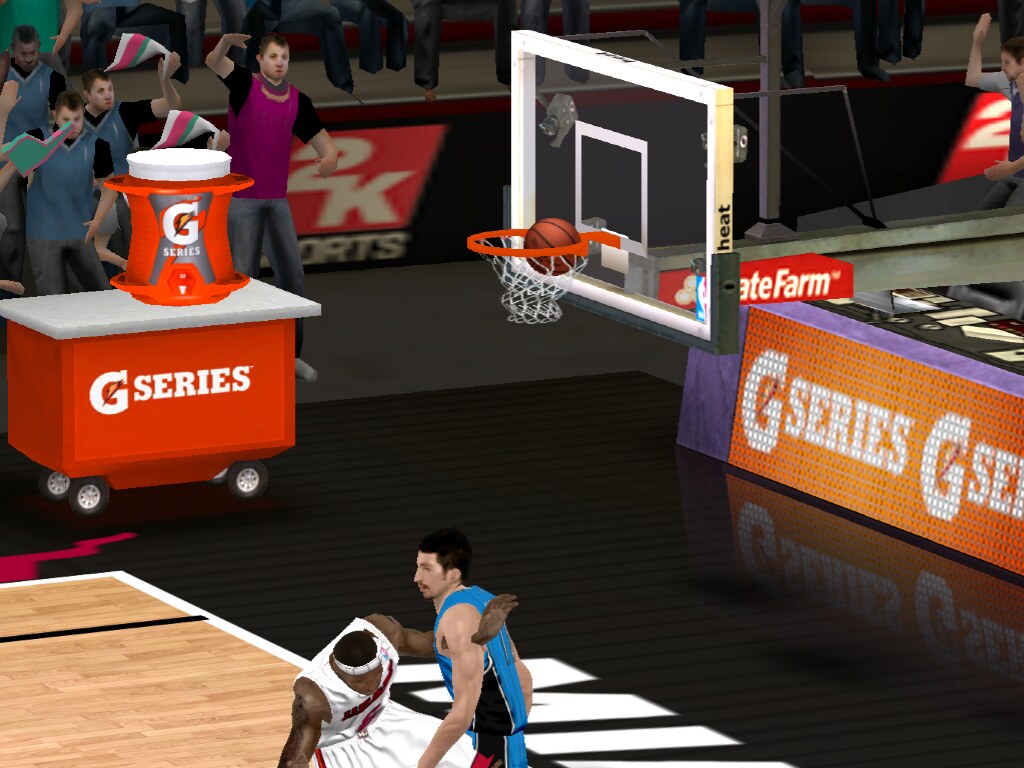This image captures a moment from a basketball video game, likely from the earlier PS4 or Xbox 360 era, showcasing impressive yet somewhat rudimentary graphics. The scene focuses on a black and gold basketball court with a section of hardwood floor visible in the lower-left corner. Centered in the frame, two players vie beneath the hoop: a light-skinned player in a blue and black jersey and shorts, and a dark-skinned player in a white and red uniform. The basketball is seen sinking into the net above them, with a noticeable visual glitch where one player's hand clips through the other. 

In the background, fans in casual attire enthusiastically cheer on the action. Advertisements punctuate the scene, with an orange and purple "G-Series" sign and a red "State Farm" sign prominently displayed around the backboard. A red cart with wheels, featuring a red Gatorade cooler, underscores the game's product placement. The immersive details and vibrant atmosphere suggest the game was ahead of its time, despite displaying some characteristic graphical limitations of its generation.